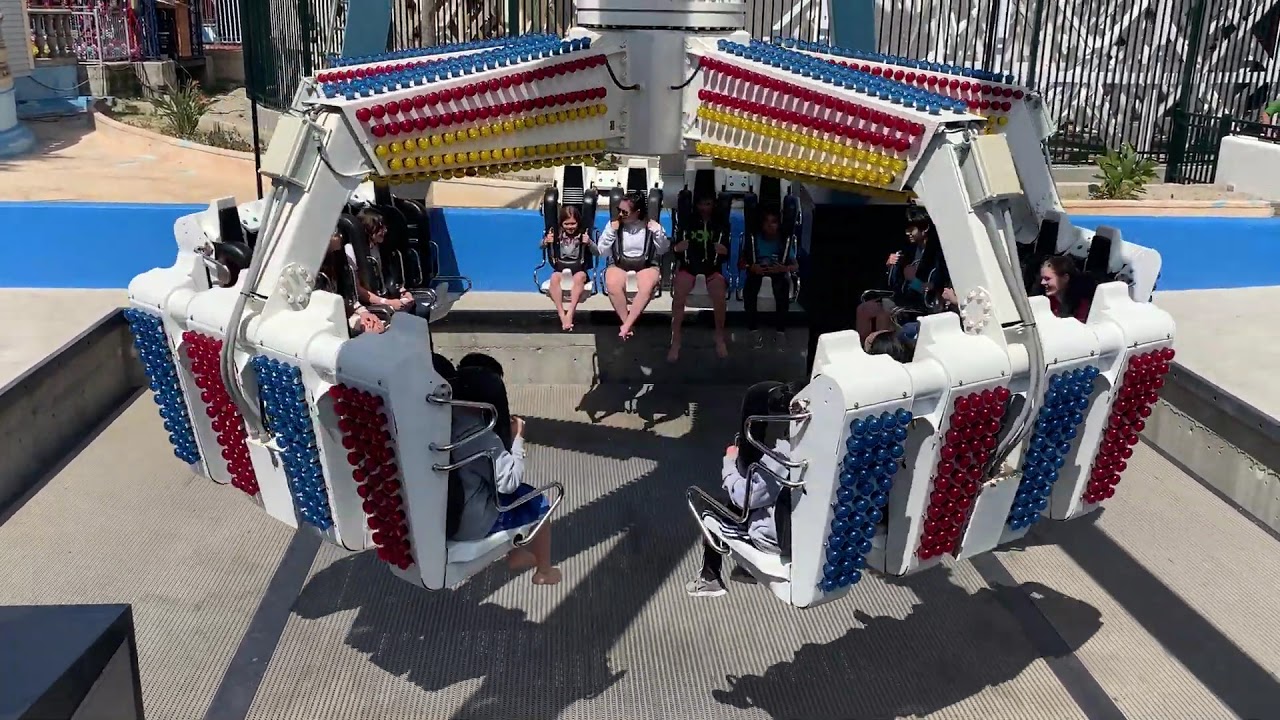The image depicts a vibrant carnival ride shaped like a giant claw, designed to seat 20 people, with five sets of four seats each, arranged in a circular layout. Each set of seats is secured to the prongs of the claw and features colorful lights—blue, red, and yellow—illuminating the backrests. The riders are strapped in with harnesses, ready for the ride to begin. The scene captures a mix of passengers, including a little girl, a woman looking at her, a man beside them, along with others filling nearly every seat. In the foreground, a girl wearing pink Crocs is visible on the left, with another individual’s legs hanging down on a separate prong to her right. The ride hovers above a gray cement ground with ridges, enclosed by a blue fence. The amusement park ambiance is further accentuated by the structural details, including metal crossbars and a central cylinder at the top, contributing to the energetic and dynamic atmosphere of the fairground.